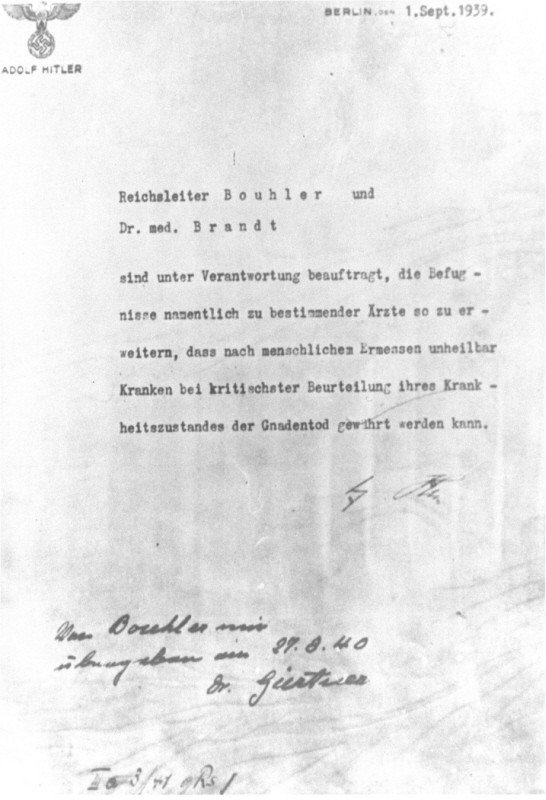The image depicts an old typewritten letter, possibly a photocopy, dated September 1st, 1939, from Berlin. The letter is linked to Adolf Hitler, evident from the top left-hand corner, which features a Nazi symbol with an eagle atop it and Hitler's name beneath. The letter, addressed to Reichsleiter Bühler and Dr. Medbranch, is entirely in German and illegible to non-German speakers. There is a signature at the bottom, alongside some handwritten notes, including a date of August 27, 1940, and some indistinguishable numerical annotations. The photo, black and white, showcases a worn document, possibly indicative of its age and the journey it has undergone.